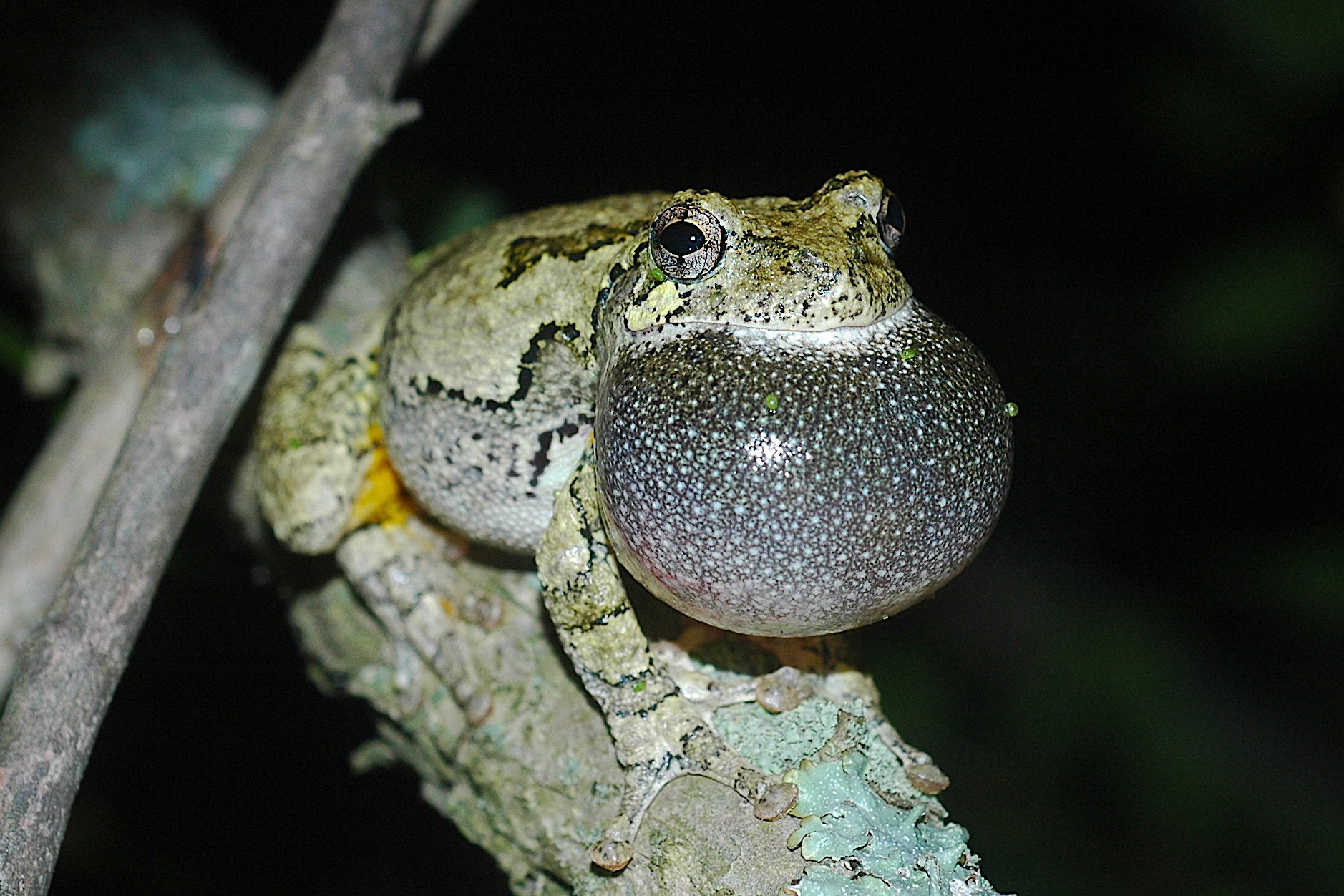This detailed photograph captures a frog perched on a tree branch at night. The background is almost entirely black, offering an exquisite contrast that highlights the frog and its surroundings, making the scene pop. The frog, an army green or olive green with distinctive black striped patterns along its face and body, is in the midst of croaking—its chin and chest expanded into a large, bubble-like shape. The expanded area showcases intricate designs with what seems to be black and white spots. The frog's eyes, big and expressive, appear to be staring off into the distance, giving it an almost introspective look. On the left side of the image, a couple of additional branches lie next to the main one, adding compositional balance to the photograph. While the specific species of the frog is indeterminate, the visual details and setting create an enthralling snapshot of nocturnal wildlife.